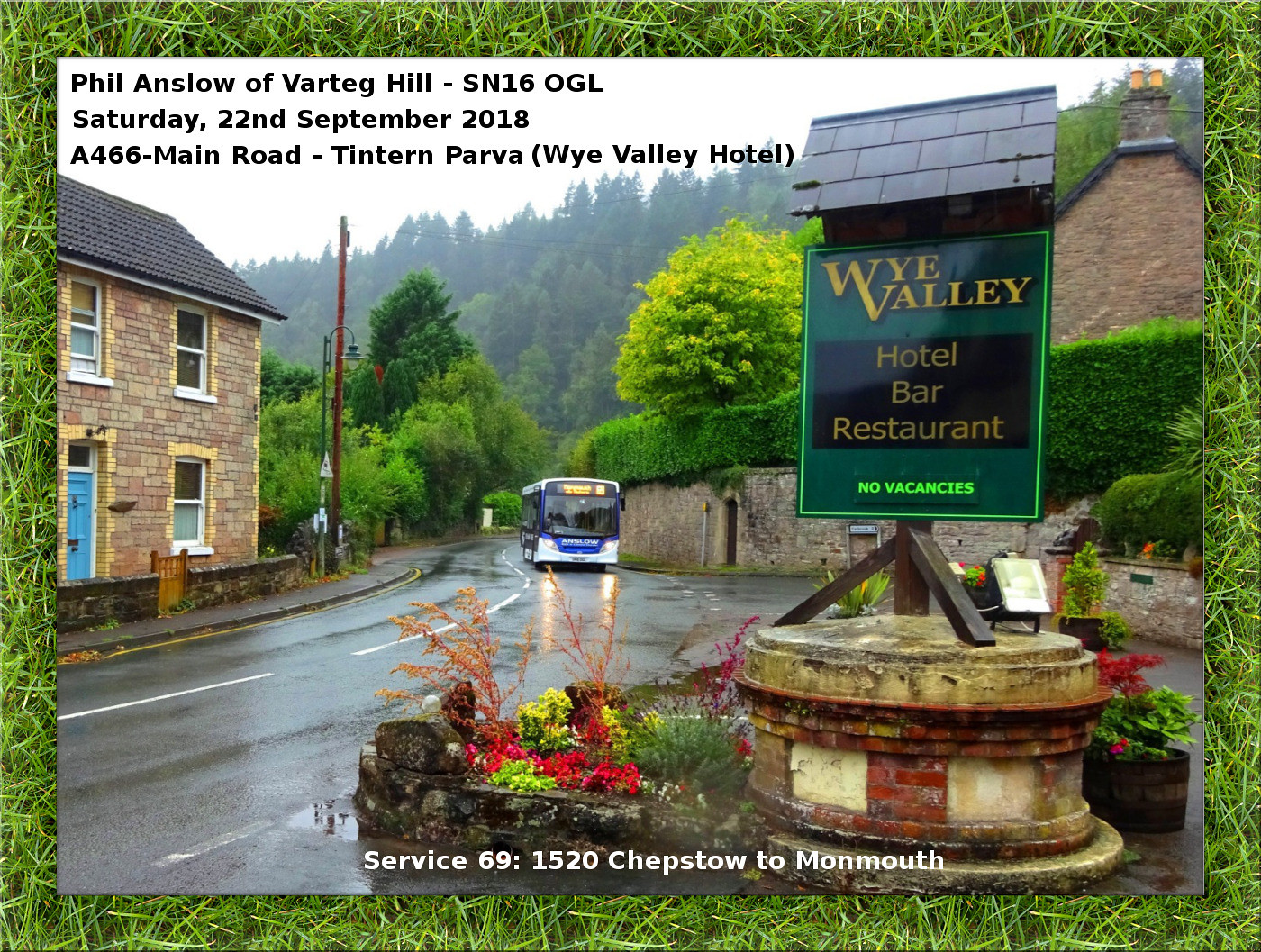The image depicts an English countryside village with a central focus on a blue and white public bus navigating a wet, curved country road. The bus is prominently placed in the center, heading through the village. On the left side of the road is a brick building with a blue door, three windows, and a black shingled roof. On the right side, there's a brick wall and a distinctive hotel and bar sign for the Wye Valley Hotel, Bar, and Restaurant, which includes details such as "no vacancies" in yellow, green, and black colors. This sign features a small roof with black shingles and is emerging from a structure covered in flowers. Surrounding the road and buildings are lush greenery and distant mountains with high-reaching trees, enveloping the scene in a verdant embrace. Additional text elements describe: "Phil Anzalo of Varteg Hill and SN 16 OGL Saturday 22nd September 2018, a four six-ish dash main road dash ten turn Parva (why Valley Hotel)", and at the very bottom, "service 69 1 5 2 0 chipstone to Monmouth" in white font. The overall style suggests an advertisement, postcard, or photograph capturing the quaint and picturesque essence of the English countryside.